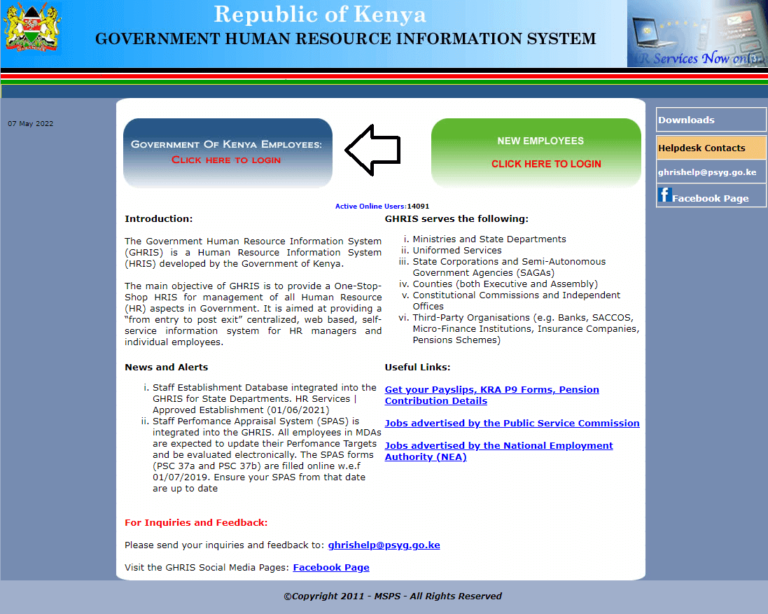The image is a square box with a blue background that features several elements associated with the Republic of Kenya's Government Human Resources Information System. At the top, a lighter blue banner displays the text "Republic of Kenya" in white letters, with the phrase "Government Human Resources Information System" immediately below it. To the left of this text, an icon appears, though its specific design is not detailed.

In the center of the image is a prominent white box. On the top left of the white box, the text "Government of Kenya Employees" is written in white letters. Below this, a blue button labeled "Click here to log in" features the instructions in red text. Adjacent to this button, an arrow points right towards another section meant for new employees. The section for new employees includes a green button labeled "Click here to log in," also in red text.

Beneath these buttons, a bold line reads "Active online users" in blue, with an active user count of 14,091. Further down, there is an introduction section containing a substantial amount of information (not detailed here), followed by a segment labeled "News and Alerts."

At the bottom of the white box, the text "For inquiries and feedback" appears in red, accompanied by an email link and a Facebook page link. To the right of the "News and Alerts" section, there is a "Useful Links" section with several blue hyperlinks.